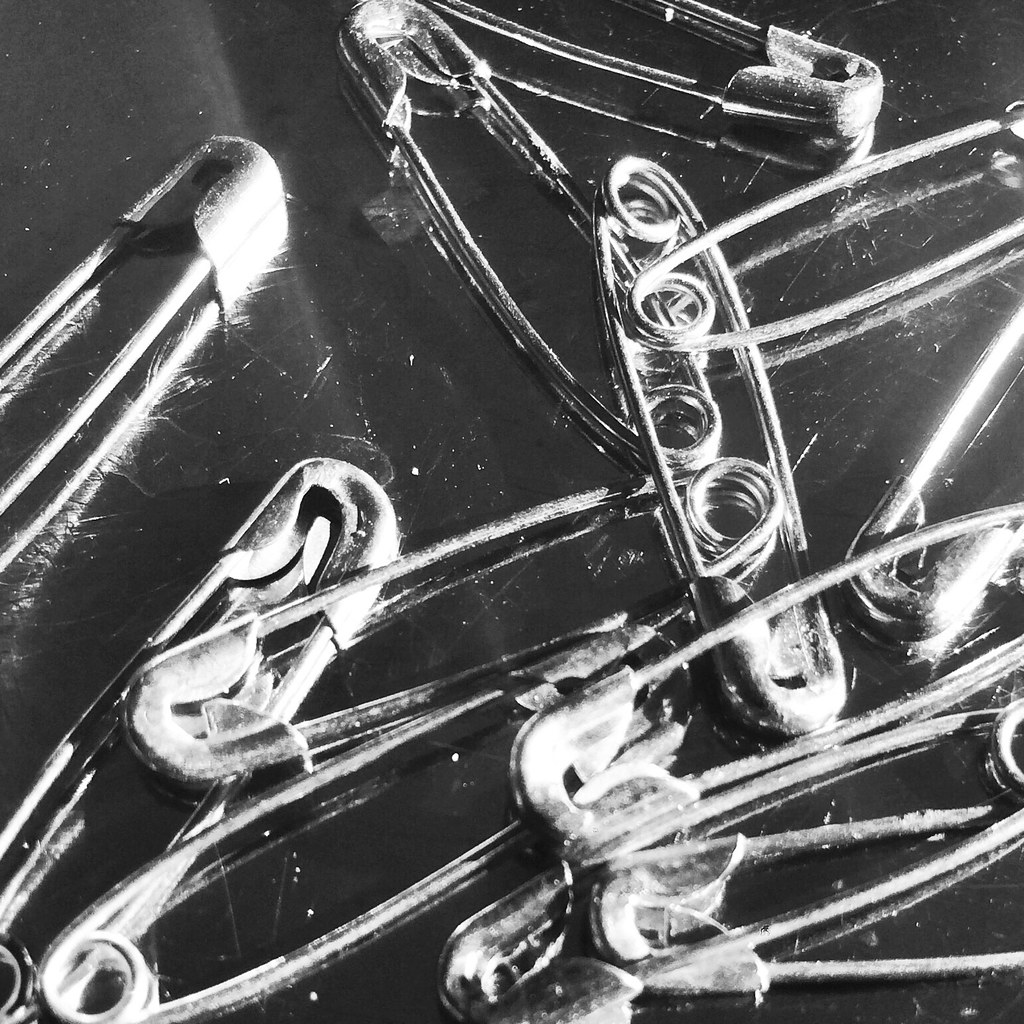This black and white photograph showcases approximately ten metal safety pins haphazardly arranged against a scratched, black background. The safety pins appear to be both black and white in color, likely due to reflective light shining from above. The top parts of the safety pins, particularly those in the upper left and lower right corners, feature white splatters and drips, which spill onto the surrounding black surface, creating an almost painted effect. Among the pins, one is distinguishably open, with its pointed end visible. Numerous white specks are scattered throughout the background, adding to the abstract composition of the close-up image.